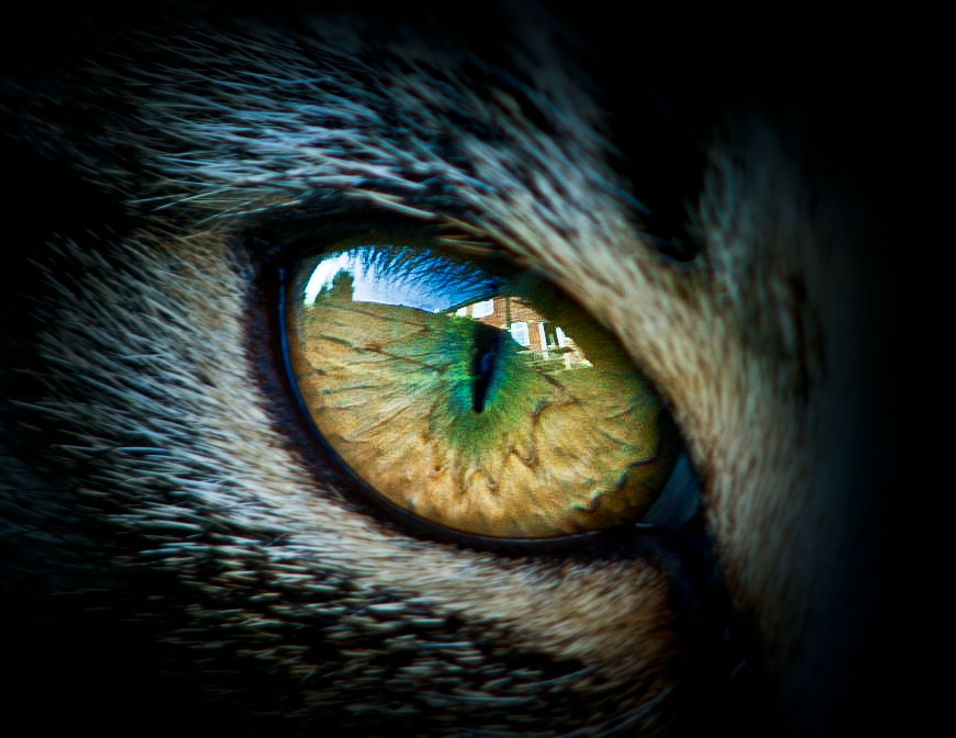This highly detailed, rectangular photograph, almost square in shape, showcases an extreme close-up of an animal's eye, likely a cat. The eye, which is central to the image and takes up most of the frame, features a slitted pupil surrounded by a gradient of colors—from green to yellow. The surrounding fur transitions from brown to gray, becoming darker as it reaches the periphery, indicating the rest of the face is cast in shadow. The eye itself reflects a vivid outdoor scene: a brick building with an open window, a blue sky, and a tree to the left. This reflection is captured crisply and clearly, adding a layer of depth and intrigue. Detailing around the eye is impeccable, revealing individual eyelashes and strands of fur. The surrounding darkened border enhances the dramatic focus on the eye, making the image both fascinating and visually striking.